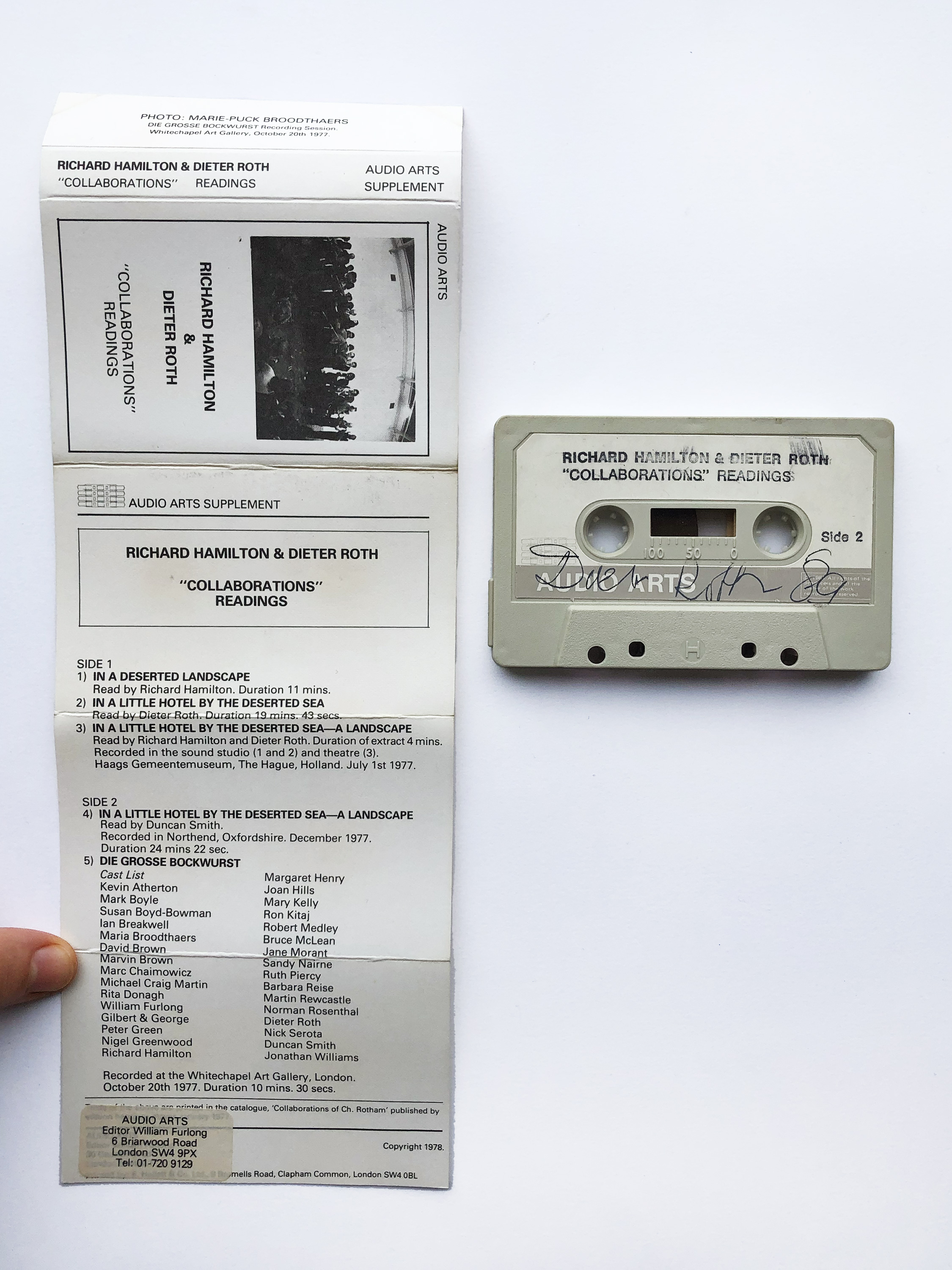This color photograph features a gray cassette tape and its unfolded white cardboard insert, both prominently displayed. The insert, occupying the left-hand side of the photograph, stretches from top to bottom and showcases a black and white cover at the top. The cover is adorned with the title "Richard Hamilton and Dieter Roth Collaborations Readings," accompanied by detailed contents in smaller print below the title, which are illegible due to their small size. To the right, the cassette tape is labeled with "Richard Hamilton and Dieter Roth Collaborations Readings" in black text on a white background. The brand "Audio Arts" is printed in white text on the cassette. A barely legible signature in black handwritten text graces the front of the cassette. Additionally, a human thumb is visible at the very lower left corner of the photograph, adding an element of human presence. The background of the image is a plain white surface, enhancing the clarity and focus on the cassette and its insert.